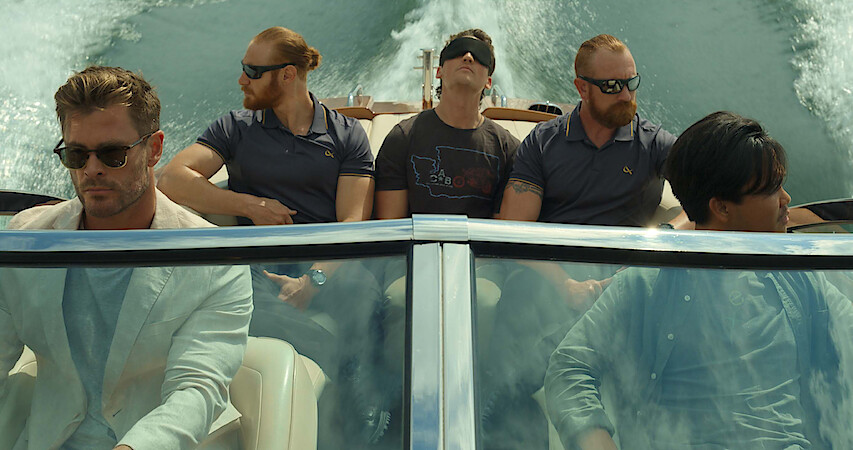The image appears to be a screenshot from a movie, featuring five men in a speeding speedboat that is creating a large wake, indicating it's moving at high speed. At the helm of the boat, on the front left, is a man with slicked-back blonde hair, wearing a white jacket over a blue shirt, and sporting gold-rimmed sunglasses. He has a short beard and mustache. To his right, another man is looking off to the left side; he has short black hair and is dressed in a green U.V.E.R. shirt over a gray T-shirt.

In the back of the boat sit three men, appearing to form a scene where two of them, who look like security guards, are escorting a blindfolded man. The central figure in the back is blindfolded, looking upward, and wearing a T-shirt with a blue outline of a map printed on it. This man has brown hair and fair skin. Flanking him are two similarly dressed men with red hair pulled back into man buns, both muscular and sporting beards and sunglasses. The man on the left is wearing a short-sleeve blue collared shirt with a gold emblem at the pocket level, while the man on the right has a sleeve tattoo and is dressed in similar attire.

The boat itself is white with brown trim and has windows lined with silver or brushed aluminum. The entire scene appears to be set during the day, with the boat cutting through cyan-colored water, leaving trails of white foam behind.